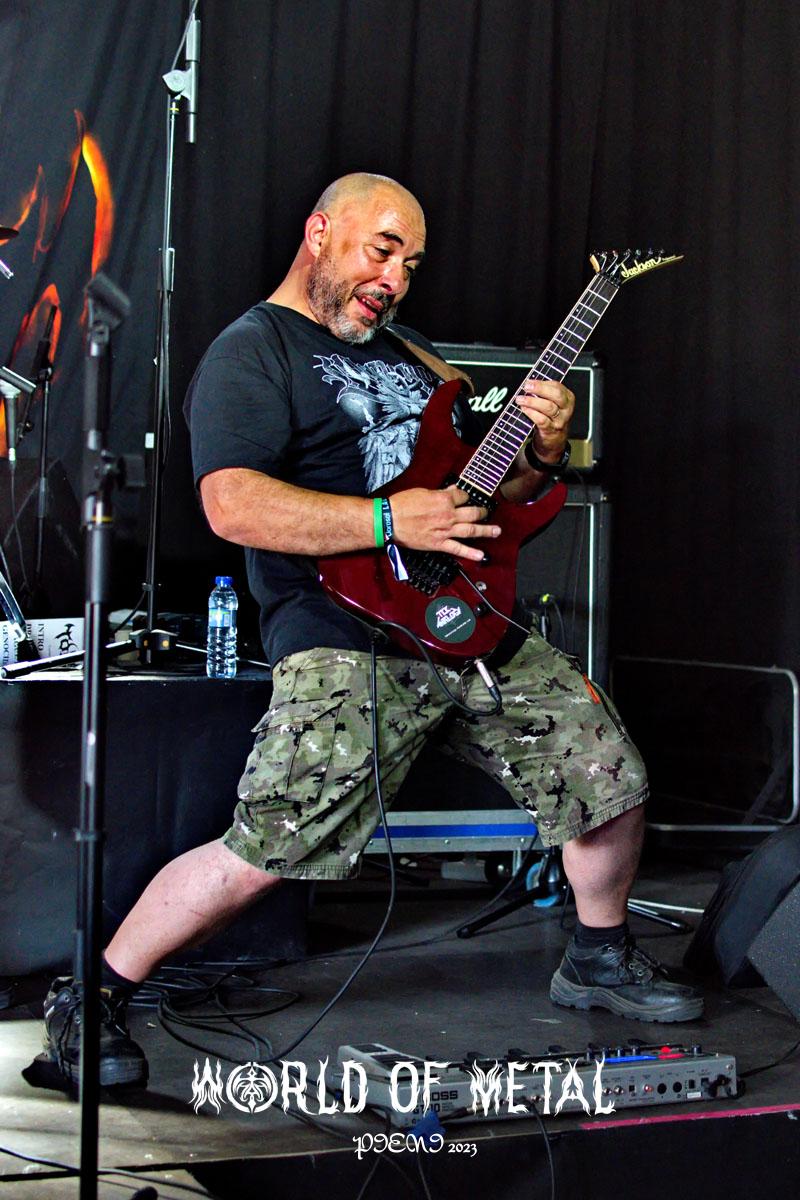In the image, a man is playing an electric guitar on a well-lit stage with a black floor. The backdrop is a black curtain, contrasting with the man's outfit and emphasizing his presence. The guitar is a dark brown Jackson brand with a black circular sticker, connected to an amplifier with a Marshall brand head. The musician is bald with a neatly trimmed dark beard and mustache, exuding a focused yet joyful expression as he performs. He is dressed in a black short-sleeved T-shirt adorned with a white and gray print on the chest, and green camouflage shorts with white and black prints. Completing his outfit, he wears black tennis shoes paired with black socks. Accessories include a black watch on his left wrist and a green wristband alongside a darker-colored bracelet with some kind of writing on his right wrist. Positioned behind him are a rolling amplifier, a water bottle, and another microphone stand without a microphone, suggesting the presence of additional equipment or band members just out of frame. A silver pedal board lies at his feet, and a wall of metal with the label "P9EN9, 2012-2023" is seen at the bottom, possibly indicating a poster or magazine title. The entire composition centers on the guitarist, highlighting his intense connection with the music and stage.